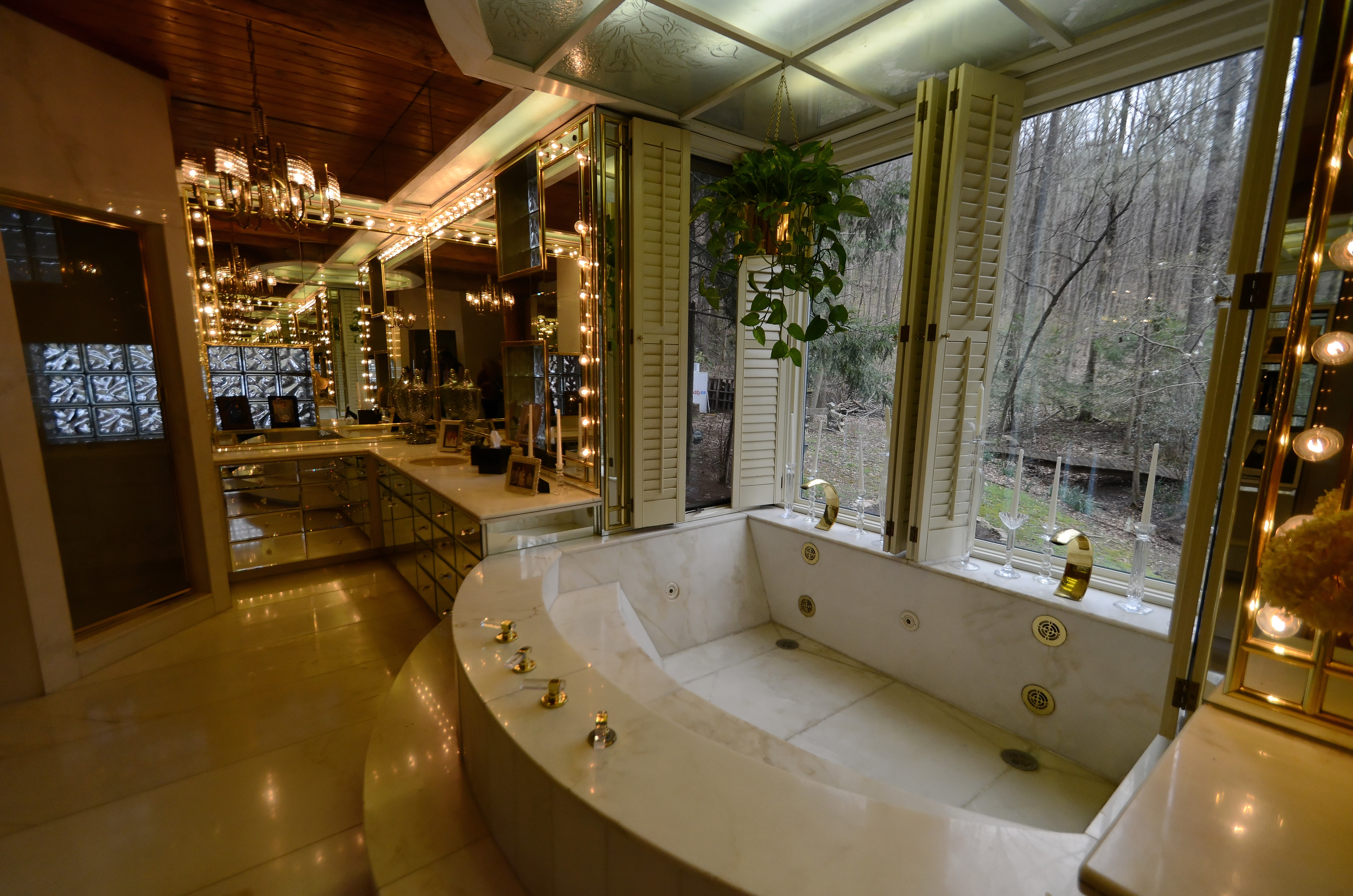The photograph displays a large and lavish bathroom, bathed in elegance and luxury. Dominating the center is an expansive marble bathtub with a unique design: three straight edges and a curved edge facing the room. The curved part is adorned with multiple gold-plated knobs, while two grand gold faucets grace the outer part closest to a pair of large windows. These windows have tan shutters, which are open, revealing a wintry or autumnal scene with trees devoid of leaves. Unlit candlesticks rest on the windowsill, adding a touch of classic charm.

On the right side of the image, a makeup table is set up, complete with a mirror encircled by multiple light bulbs, creating a bright and glamorous focal point. Below the mirror, there are cabinets that appear to be gold-plated, enhancing the opulent feel. The flooring throughout this sumptuous space is a pristine white marble, reflecting the luxurious ambiance. The overall atmosphere is one of splendor and refinement, with gold fixtures and marble surfaces contributing to the bathroom's majestic appearance.